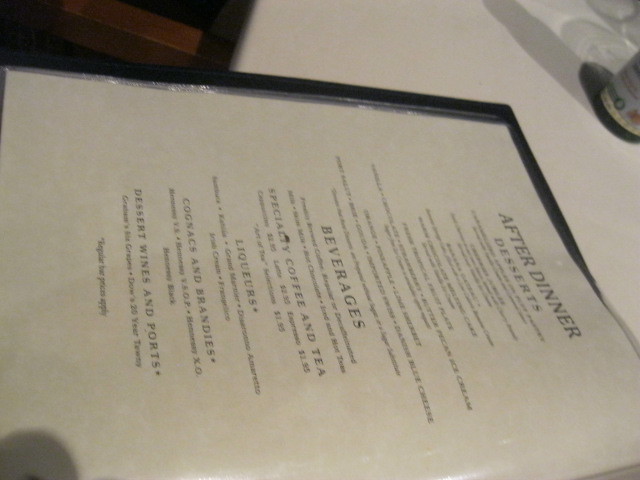A menu is placed on a tan-colored table, turned sideways, presenting a challenge to read. The top section of the menu, adorned with all-capital letters, boldly declares "AFTER DINNER," followed by "DESSERTS." While the list of desserts beneath remains illegible due to the tiny font, the structure of the menu continues methodically. Next, "BEVERAGES" appears in large capital letters, likely accompanied by a list of drink options in minuscule print. The segment below that reads "SPECIALTY COFFEE AND TEA," in smaller capital letters, presumably outlining various coffee and tea choices. Following, the word "LIQUORS" in similar-sized font denotes another category, likely listing different liquors. Further down, "COGNAC AND BRANDY" is written in the same style, suggesting a selection of these spirits. The final section features "DESSERT WINES AND PORTS" and beneath it, an indiscernible list and some italicized text. The menu is bordered in black. Adjacent to it is a dark object, partly visible but unidentifiable, with blurry background elements including a round item with lettering—potentially a can. The background is mostly distinguished by ambiguous shadows, hinting at unseen objects casting them.